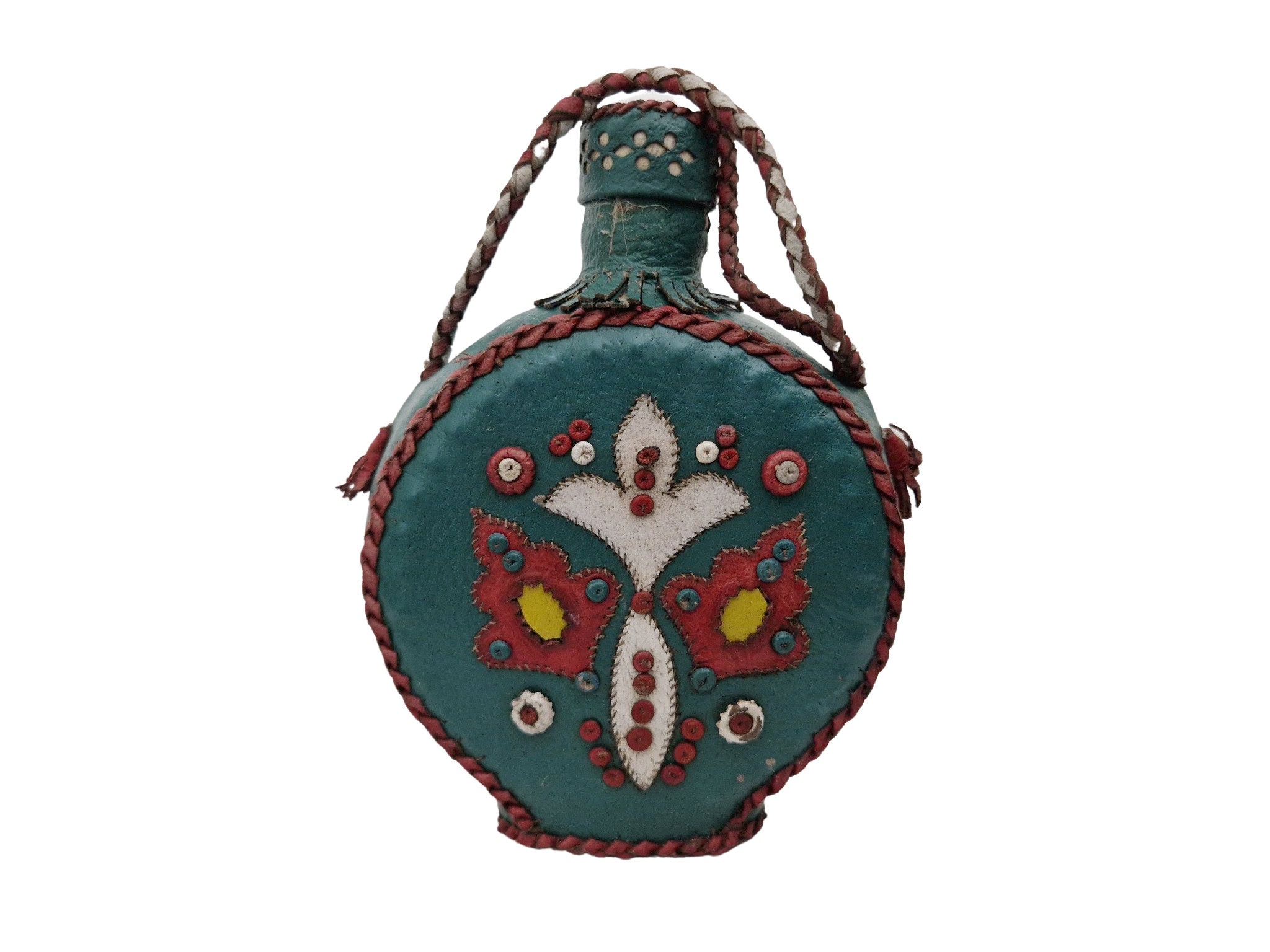The image features a striking, antique canteen, possibly inspired by or belonging to Native American culture. It boasts an intricate leather covering, meticulously stretched around the canteen in a manner reminiscent of drum construction. The leather is predominantly a dark hunter green, adorned with vibrant red, white, and gold decorative patches and intricate stitching. The front of the canteen showcases beautifully embroidered flower designs, along with button-like decorative elements. A braided handle, interlaced with red and white strands, is attached for easy carrying and adds to the traditional, handcrafted feel of the object. The top of the canteen is affixed with a removable cord, and the entire piece exudes the charm of folk art, suggesting that it is a unique, handmade item rather than a mass-produced product. The canteen is presented against a plain white background, highlighting its detailed embellishments and rich cultural heritage, which gives it an appearance suitable for display in a museum.